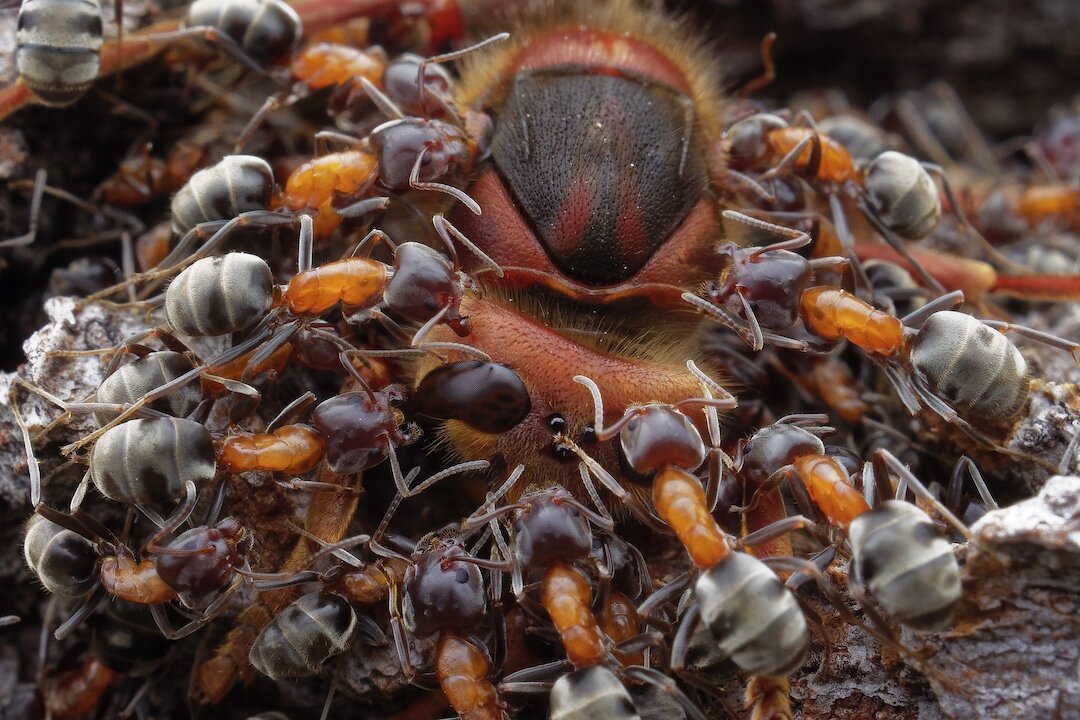This detailed, macro-style, color photograph in landscape orientation captures a dramatic scene of a large orange-and-black spider being besieged by a coordinated swarm of sizable ants. The ants, characterized by their distinctive dark red, semi-transparent heads with black eyes and dual antennae, display a vibrant gold thorax and a gray-and-black striped abdomen. These ants, nearly resembling wingless wasps due to their size and translucent body parts, are seen ferociously attacking the much larger orange spider, which features a central black triangular marking and yellow hairs along its body. The spider's striking black shield-like marking, adorned with two red spots at the base, adds to the visual intensity as the surrounding ants, clamping with their red pinchers, seem poised to move their oversized prey. The photograph's realism and close-up perspective draw attention to the intricate details of the ants' aggressive interaction with the spider.